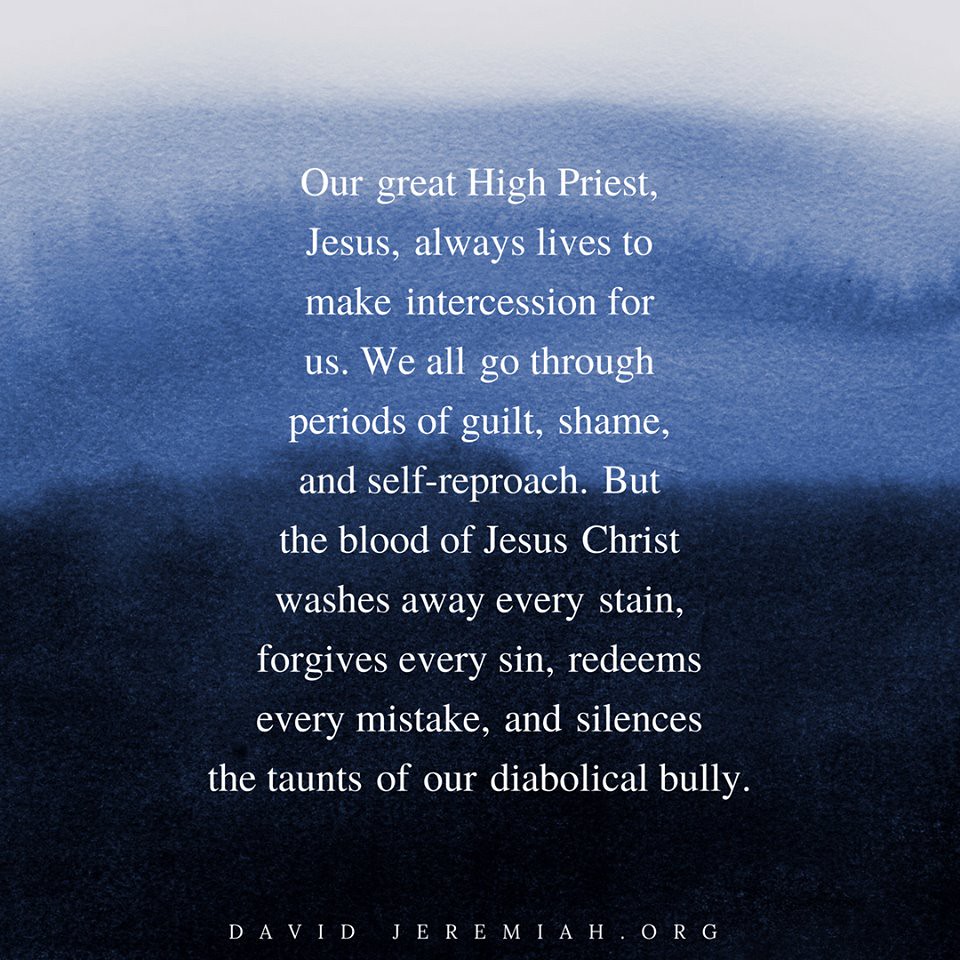The image is a square-shaped poster featuring a quote in white text over a blue background that transitions from light blue at the top to a darker blue at the bottom. The background appears to have a blurry, wave-like texture, possibly with faded mountains, enhancing the ethereal feel of the design. The quote reads: “Our great High Priest, Jesus, always lives to make intercession for us. We all go through periods of guilt, shame, and self-reproach, but the blood of Jesus Christ washes away every stain, forgives every sin, redeems every mistake, and silences the taunts of our diabolical bully.” The source of the quote, "DavidJeremiah.org," is prominently displayed in uppercase letters at the bottom of the image.